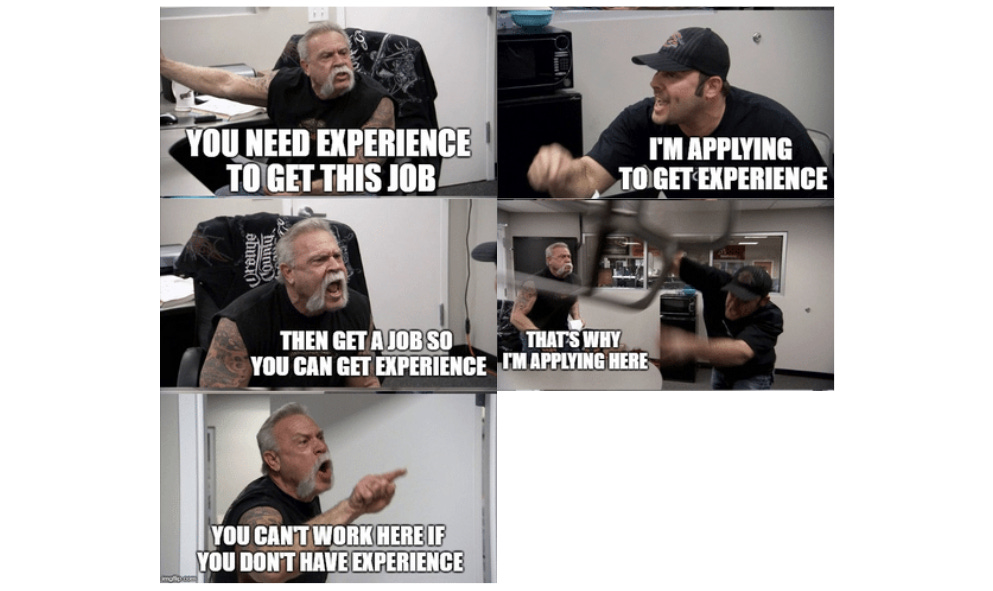The meme consists of a sequence of five small pictures arranged vertically, depicting an increasingly frustrating conversation between an older man and a younger man about the paradox of needing experience to get a job. In the initial frame at the top left, an older man with long white hair, a white mustache, and wearing a sleeveless shirt, sits in a desk chair, extending his right arm while yelling, "You need experience to get this job," in bold white capital letters. To the right, a younger man in a black short sleeve shirt and black baseball cap, also yelling, replies, "I'm applying to get experience!" in similar bold white caps. The second row begins with the older man still yelling, his arms now down in front of him, and labeled with, "Then get a job so you can get experience." To the right, both men are standing with the younger one appearing to dodge something thrown at him, stating, "That's why I'm applying here!" In the final frame on the bottom left, the older man is standing and pointing angrily against a white wall, concluding with, "You can't work here if you don't have experience." This image humorously yet frustratingly illustrates the common job-seeker's dilemma where gaining required experience becomes a circular and seemingly impossible task.